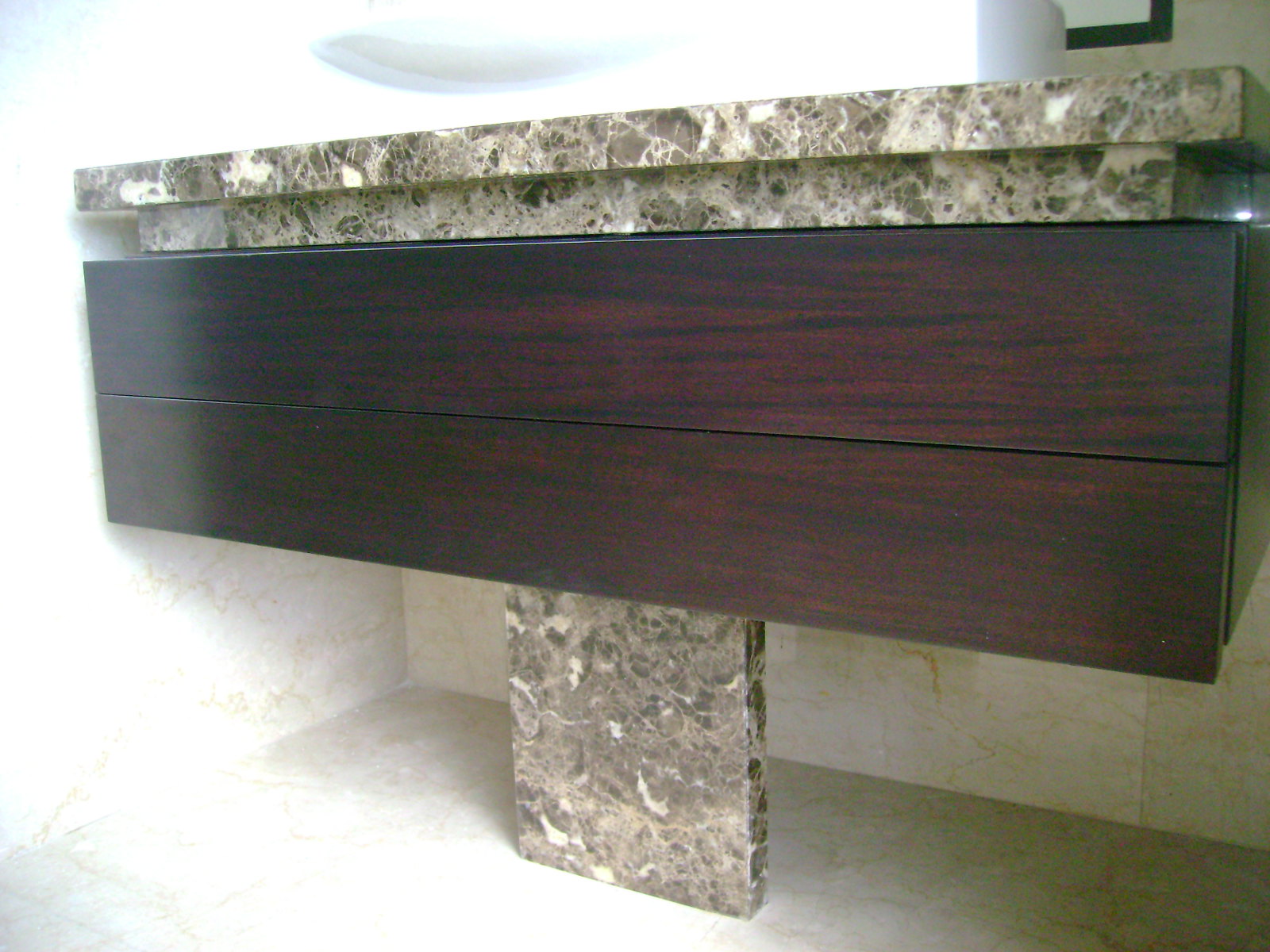The image showcases a sophisticated design of a table or counter, combining luxurious marble and rich, dark cherry wood. The structure features two horizontal pieces of wood, each exhibiting a distinct horizontal wood grain. These wooden elements are stacked vertically, creating a dynamic layered appearance. The base of the table is crafted from marble, which is seamlessly echoed at the top of the wooden sections, enhancing the cohesive aesthetic.

Surrounding the table, the floor and walls are also clad in marble, providing a continuous and opulent backdrop. On the right edge of the countertop sits a coffee cup, adding a touch of everyday life to the scene. The photograph is brightly lit from above, casting pronounced shadows below the counter, highlighting the interplay of light and materials in the space.